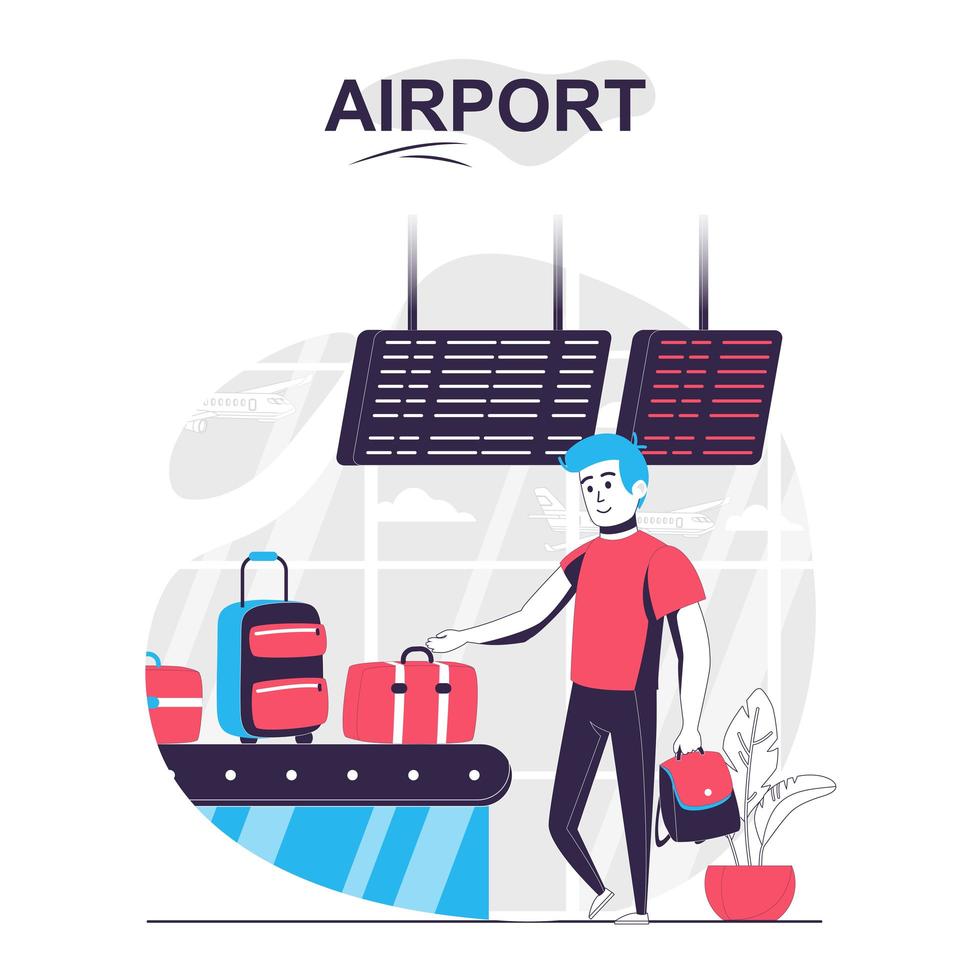This image is a detailed clip art advertisement for an airport. The background is entirely white, with a cloud-shaped, grayish figure at the top featuring the word "airport" in bold black lettering. Under this, a thin black line stretches across with another shorter line beneath it. Below these lines, there's an airport scene encased in a circular gray blob shape.

The scene showcases a man standing and facing to the left, dressed in a red shirt, black pants, and white shoes. He has distinctive blue hair and wears a black choker. His right hand is reaching to pick up a red-striped suitcase from a black conveyor belt with a blue base. The suitcase has red and white stripes and features two black dots and a black handle on the front. In his left hand, he holds another black bag topped with red.

Beside him stands a potted plant with a red half-circle pot containing white leaves. There is also a blue roller bag with a black handle extended up, positioned near a red toolbox-like briefcase. Behind the man, the background illustrates an airport setting, featuring large windows showing a gray sky with white clouds and a white airplane.

Two suspended screens hang from the ceiling, one large rectangular black screen with white slits, held by two poles, and another smaller black box with red slits held by a single pole. These evoke the typical airport display boards that show flight information.